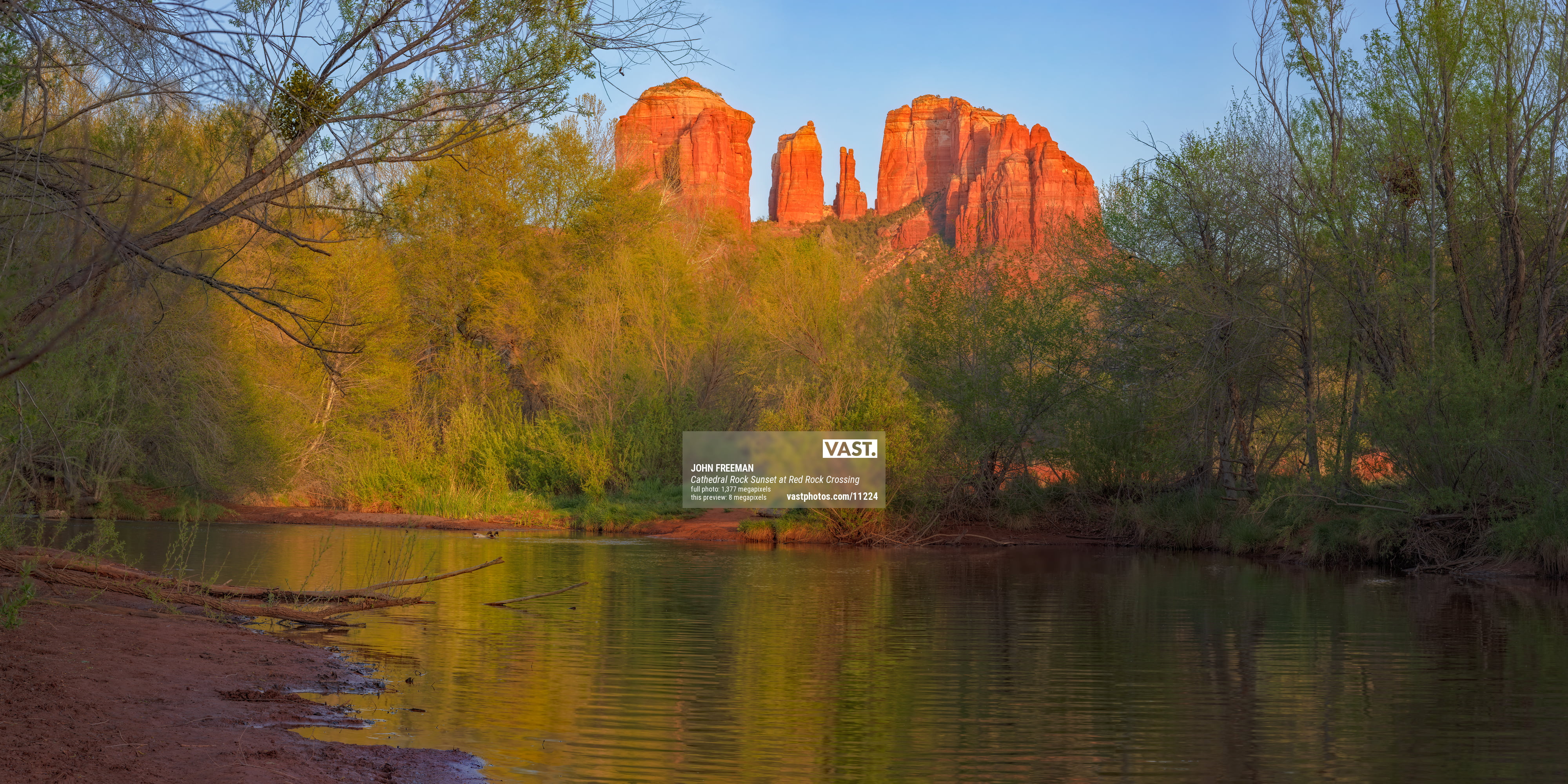The outdoor scene captures a serene body of water surrounded by green, deciduous trees in their spring bloom. Beyond the trees, the bright orange-red peaks of a mountain range rise dramatically, their unique rock formations catching the brilliant daylight. A clear, light blue sky frames the mountainous backdrop. The vivid orange hue of the mountains is so intense, thanks to the sunlight, that it is reflected beautifully in the green-tinged water of the small pond. The water's edge features a large, gray sign that prominently displays the word "vast," though additional, smaller lettering and a possible website below are not entirely legible. This picturesque scene combines the natural elements seamlessly, with the tranquil pond in the foreground and the towering, colorful mountains punctuating the horizon.